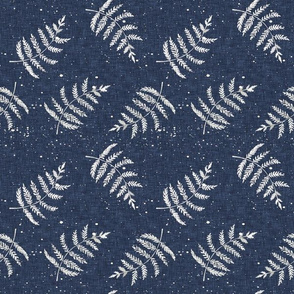The image showcases a textile or wallpaper pattern with a repeated design of detailed and delicate white fern leaves, each featuring prominently defined veins. These leaves are arranged in rows of mirrored images across a square layout, positioned uniformly at the same angle and distance from one another, creating a naturalistic and calming effect. The background is a dark navy blue with a textured, fabric-like appearance, subtly mottled with small, lighter specks that add depth and complexity. Each fern leaf comprises seven pairs of side leaves, forming a symmetrical triangular shape with a tiny leaf at the top and a visible stem at the bottom. This intricate, yet simple pattern stands out vividly against the rich, textured background, producing an elegant and soothing visual experience.